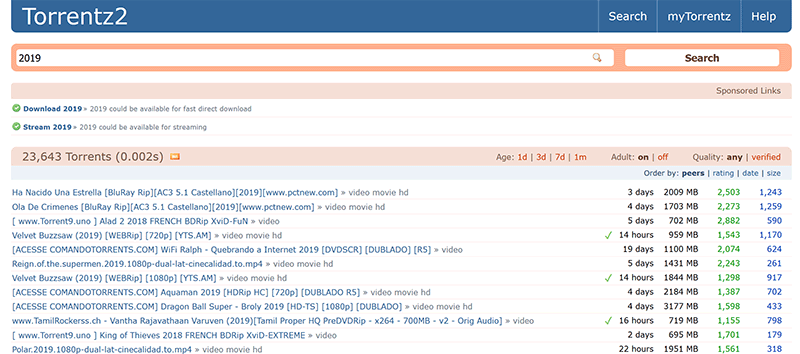This image, sourced from a website, features a layout with a prominent, long, and slender bluish-gray rectangle at the top, showing "Torrents 2" written as "T-O-R-R-E-N-T-Z 2" on the upper left-hand side. Moving toward the right side within the same header area, it includes links labeled "Search," "My Torrents," and "Help." Below the "Torrents 2" title, there is a date indication marked for the year 2019. At the far right end of the header, there is an additional search bar aimed at providing further search functionality.

In the central section of the image, large text reads "Download 2019" and "Stream 2019," indicating available download and streaming options for content from 2019. Beside these messages, additional text notes that 2019 content could be available for fast direct demand and streaming services.

Finally, the lower section of the image contains various comments and entries, organized into multiple columns, each detailing different information with some entries spanning several days. The structure suggests a forum or discussion-like section dedicated to user interactions and content indexing.